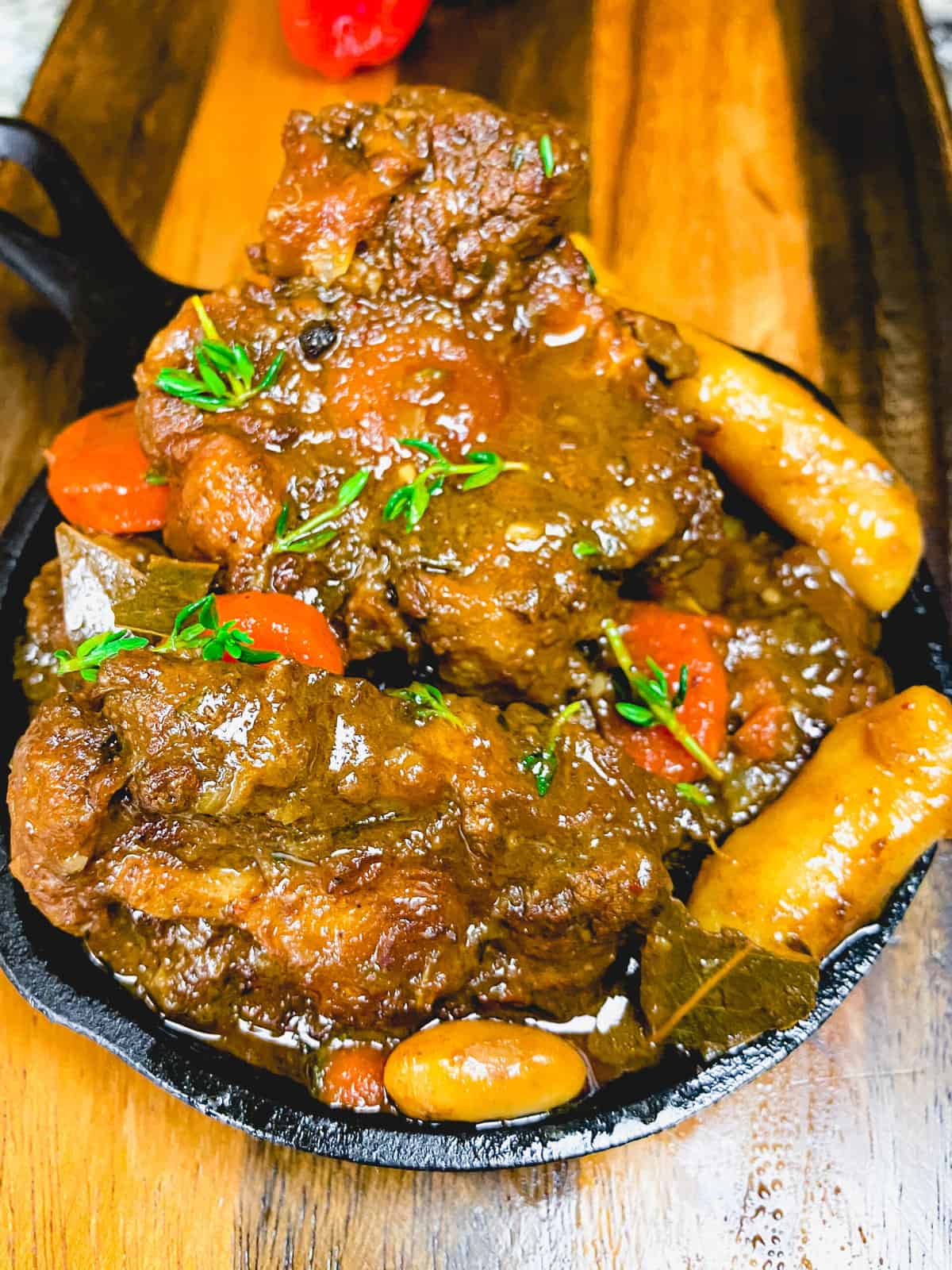This image is a detailed, portrait-style color photograph capturing a savory, towering dish generously piled inside a cast iron pot. The dish consists primarily of substantial, chunky beef pieces cloaked in a rich brown gravy, accompanied by sizable carrot slices and fingerling potatoes. Fresh green garnishes sprinkle the top, adding a vibrant contrast to the hearty meal. The stew-like concoction reaches an impressive height within the pot, almost to the point of overflowing, with the chunks seemingly supporting each other in a distinct structure. Two long, orange mini sausages are visible on the right side, adding further texture and color variety. The pot's handle is oriented to the left, and the entire setup rests on a light and dark brown cutting board. In the background, atop the cutting board, lies a red chili pepper, adding a final dash of color and hint of spiciness to the scene. The dish exudes a tempting aroma and visual appeal, suggesting influences from Indian or Moroccan cuisine, and is presented on a rustic, black, handmade plate. The overall setting is further grounded by the wooden beam that underpins the cutting board, enhancing the homey, culinary ambiance.